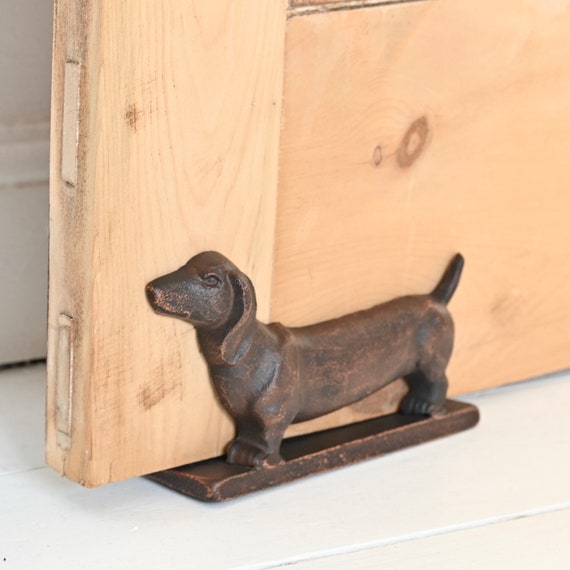This image features the bottom portion of a brown wooden door, highlighted by the detailed textures and knots in the wood. The door rests upon a floor of pristine white tile. Central to the image is a doorstop in the form of a dachshund, poised to the left. This intricately detailed dachshund doorstop, resembling heavy bronze or dark iron, showcases characteristic features such as a lifted tail, flopped ears, and the elongated body typical of the breed. The dog is mounted on a flat, dark base that slides partially under the door, indicating its functional role in holding the door open or closed. The background features a small segment of wall with white woodwork visible in the upper left corner, adding to the composition's overall balance and clarity.